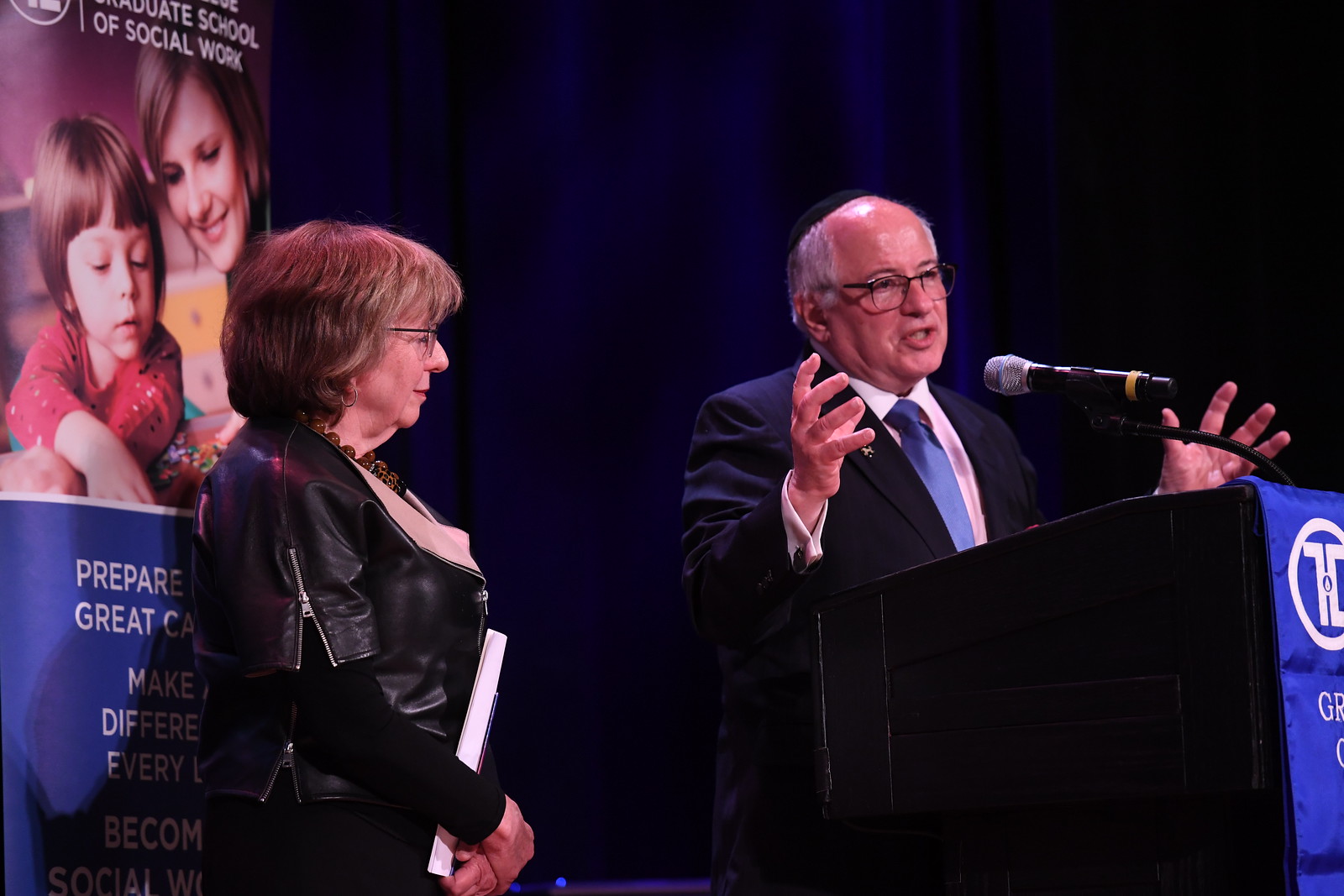This photograph captures a distinguished older man, possibly in his 60s or 70s, delivering a speech from behind a podium adorned with a blue banner featuring white text. The speaker, who appears to be Jewish as indicated by his yarmulke, has gray hair, a bald top, and glasses. He is dressed in a dark suit, white shirt, and blue tie, and is animatedly raising both hands as he speaks into the microphone extending from the podium.

To his left stands an older woman, also in her 60s, wearing a black jacket and dress, accented by a gold necklace. She has short brunette hair and glasses, and is holding a book or documents close to her chest. Behind her, a banner partially obscured by her figure reads "Graduate School of Social Work." The text visible on the banner includes phrases like "Prepare," "Great," and "Care," alongside an image of a woman and child, set against a blue background. The setting is completed by a blue curtain framing the scene behind them.